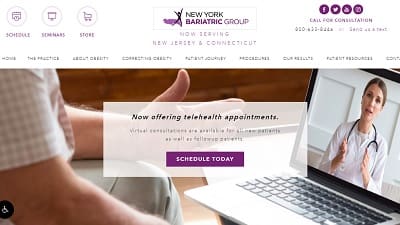The webpage depicted belongs to the New York Bariatric Group. The group's name is prominently displayed at the center top of the page. On the far left corner, there is a circular icon featuring a calendar, accompanied by the text "Schedule". Much of the textual content on the page is blurry and challenging to decipher. 

At the top right corner, several small icons are visible, likely representing social media platforms such as Facebook and Twitter, although two of the icons are indiscernible. Beneath these icons, it says "For Consultation," followed by a phone number, though the rest of the text is not legible.

Just below the header section, there is text that reads "Hours" followed by more text that is not readable due to blurriness, listing different options. 

Dominating the page is a large image that stretches the full width. The picture is a close-up of a seated man, partially showing his arms. He wears a short-sleeved check shirt, with his left hand visible in the background. His right hand would be in the foreground if visible. 

On the far right of the frame, the man is engaging in a video call via a laptop, which displays an image of a woman in white attire with a stethoscope around her neck, indicating she is a healthcare professional. The laptop keyboard is also visible. 

Overlaying the image is the text "Now Offering Telehealth Appointments - Schedule Today." This comprehensive layout and imagery communicate the group’s engagement in providing remote health consultations.